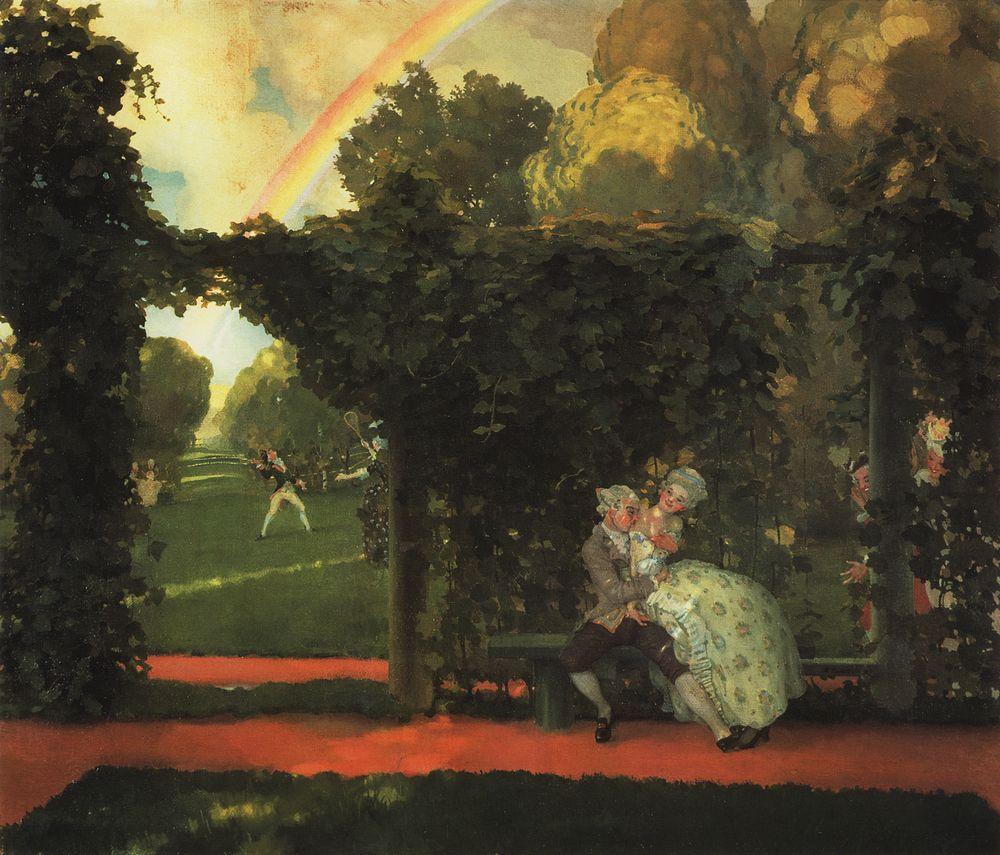In this vibrant, slightly cartoony painting of a courtyard scene, a man and woman dressed in Victorian-style clothing are seated on a bench against a garden wall adorned with lush, cascading ivy. The man, clad in a gray blazer, cover jacket, black knickers, and high white socks, tenderly pulls the woman, who is dressed in a white, poofy dress with a corset and a black hat, close as he kisses her chest. Her hair is big and fluffy, reminiscent of the grand hairstyles of the era. The scene is lively and detailed, with people dressed in similar colonial attire playing a racket sport, likely badminton or possibly lacrosse, in a field visible through an ivy-covered archway. Laughter can be seen among those observing the intimate couple. The painting's background features trees that almost blend into clouds and a radiant rainbow stretching across the sky, adding a whimsical touch to the nostalgic tableau. The pavement beneath the bench and around the garden is orange, contrasted by the surrounding green fields, flowers, and bushes.